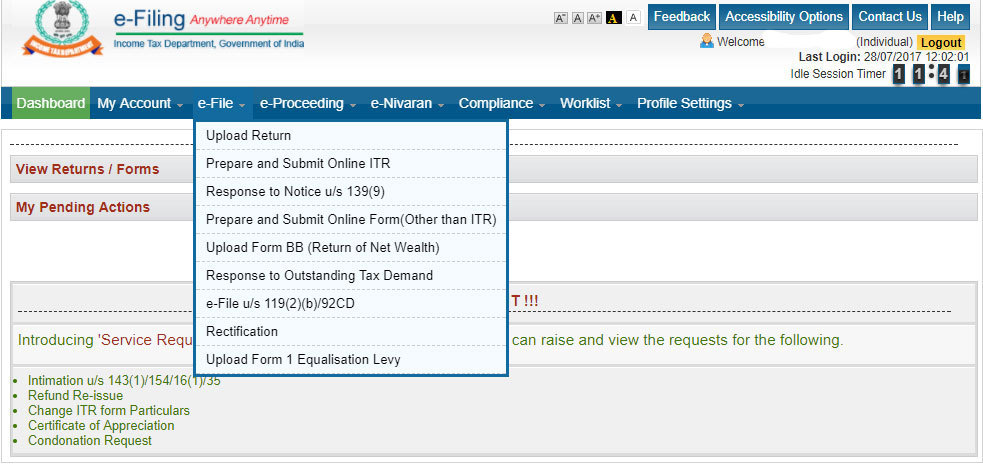This screenshot displays the homepage of the official e-filing website of the Income Tax Department of the Government of India. The topmost section features a prominent blue header with white text that reads "Income," "E-Filing," and an adjacent red text slogan stating "Anywhere Anytime." Just below this banner, it reads "Income Tax Department Government of India," indicating the authoritative source of the website. 

To the left of this text, a logo representing the Income Tax Department is visible, further authenticating the page. The main section of the page has a predominantly white or light gray background, providing a clean and uncluttered interface. A horizontal blue navigation bar stretches across the screen, featuring clickable tabs that direct to various sections such as Dashboard, Account, E-Filing, E-Proceeding, E-Nivaran (a grievance redressal system), Compliance, Worklist, and Profile Strategy. 

Below the navigation bar, there are blue buttons with white text for essential functions like contact information and help, making it user-friendly and accessible. This interface is designed to streamline the process of filing taxes, offering users multiple options to manage their tax-related activities seamlessly.